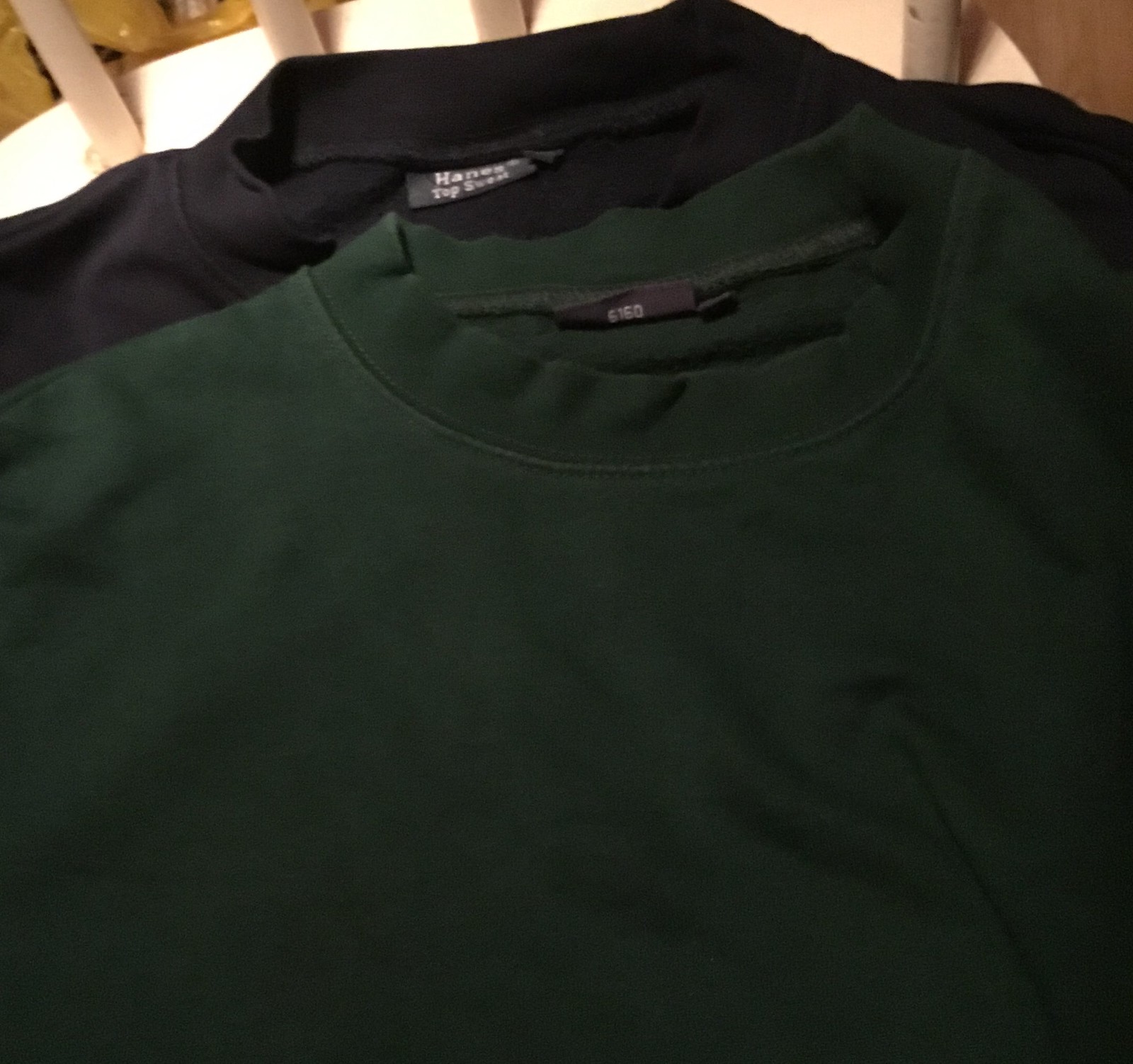The image is a close-up of two high collar style t-shirts, both layered on a wooden kitchen chair. The t-shirt on top is a dark forest hunter green, displaying its tall, thick collar and partially visible chest area. The green shirt's tag is folded, revealing the number "6160" in white on a black background. Beneath it lies a black t-shirt of the same style, also possessing a substantial collar. You can see its collar and a small part of the shoulder, along with a black tag that has the Hanes logo and some white text. The backdrop of the image includes the chair's wooden seat and vertical slats, with a glimpse of a yellow plastic bag with black writing in the upper left corner.